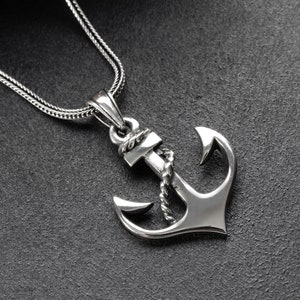The image showcases a well-lit, professionally photographed silver necklace against a dark charcoal gray, rough-textured background. The pendant of the necklace is shaped like a symmetrical ship's anchor, polished to a shiny, reflective finish. The anchor features a silver rope intricately wrapped around its body, extending towards its pointed prongs. The chain of the necklace, delicate yet not overly thin, appears braided and also made of silver. The chain emerges from the top left corner of the image, guiding the eye to the beautifully crafted anchor in the center, which stands out as the focal point of this artistic composition.